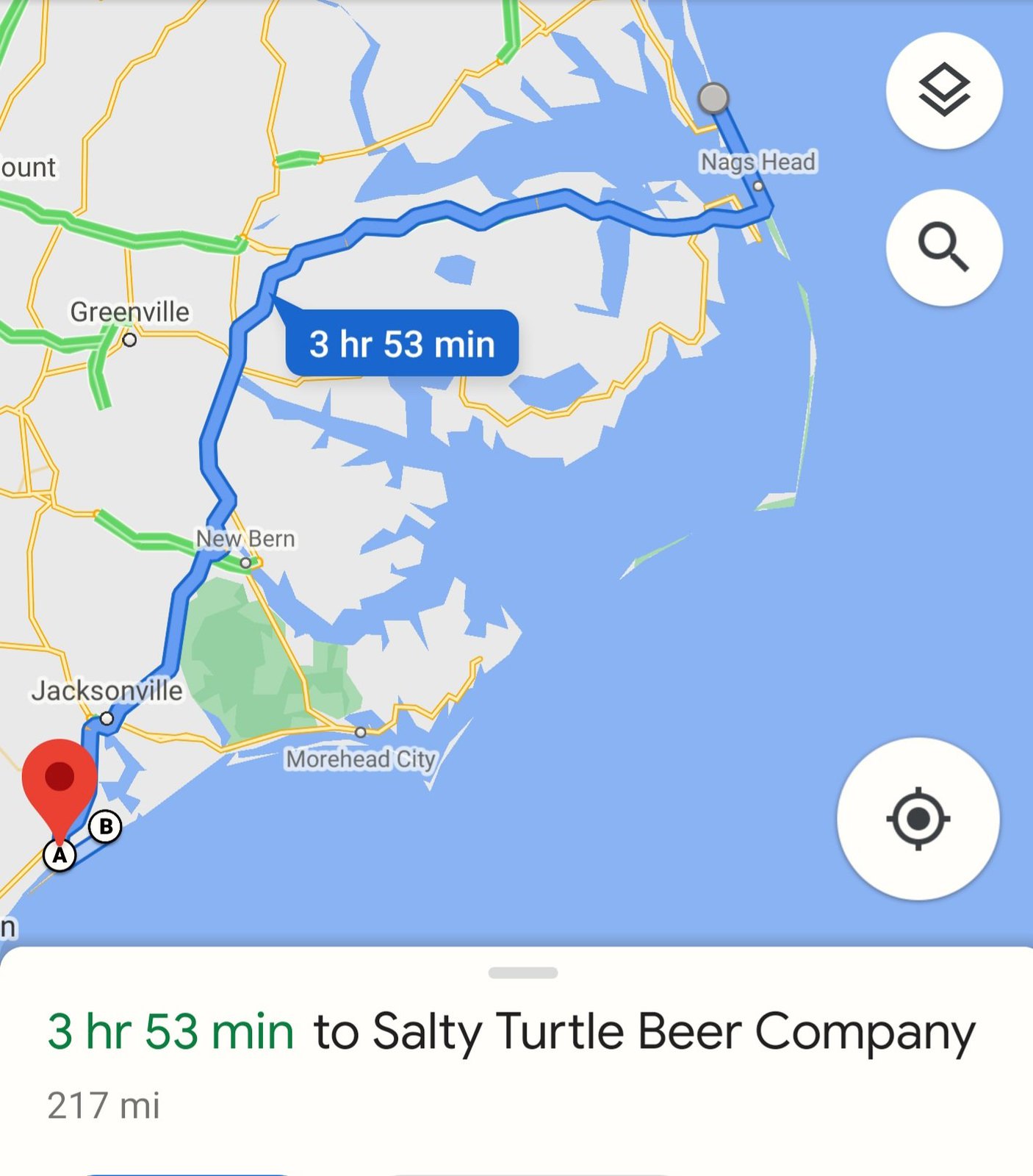The image depicts a simplified linear map illustrating the route from Jacksonville to Nags Head, a coastal destination. The map prominently features a balloon-shaped arrow indicating a travel time of three hours and 53 minutes to Nags Head. Other nearby cities such as Greenville, New Bern, and Morehead City are also marked along the route. The right side of the map is shaded blue, representing the adjacent open water of the coastline. At the bottom, a white balloon highlights additional details: the route covers 217 miles and leads to the Salty Turtle Beer Company, with the same travel duration of three hours and 53 minutes.